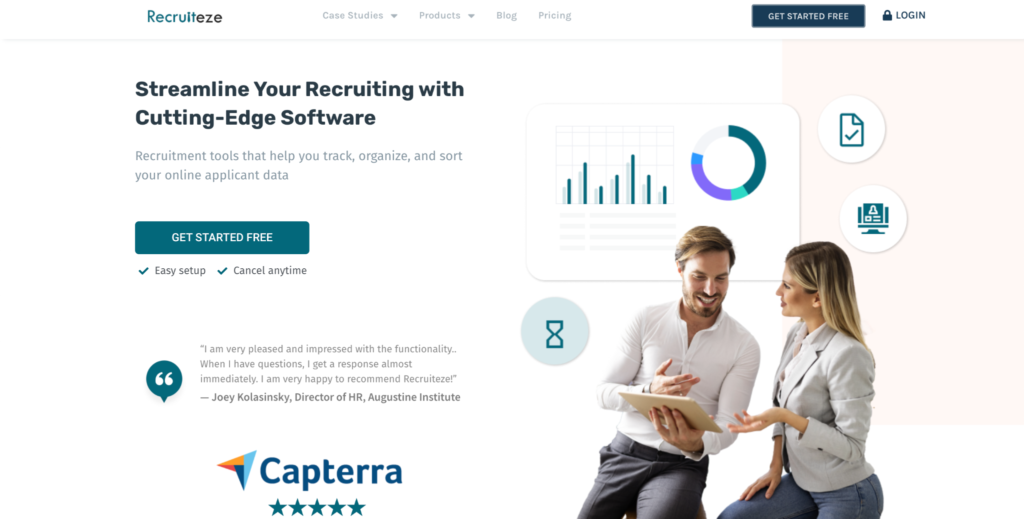The image portrays a sleek and modern webpage landing screen for an advanced recruitment software platform named "recruitEZ." The header of the page prominently features the product name "recruitEZ," with the term "recruit" in blue and "EZ" in black. Directly below the header, there is a navigation bar offering four grayed-out options: "Case Studies" with a dropdown menu, "Products" with another dropdown, and "Blog" and "Pricing," which do not feature dropdown menus. On the far right of this navigation bar, a prominent blue button displays "Get Started Free" in white text, accompanied by a "Login" button featuring a lock icon.

Beneath the navigation bar, a bold and clear message reads, "Streamline your recruiting with cutting-edge software." In smaller, lighter grey text underneath, it states, "Recruitment tools that help you track, organize, and sort your online applicant data." An additional "Get Started Free" link appears below this tagline. Further down, two checkmarks note the benefits of the service: "Easy setup" and "Cancel anytime."

A testimonial from Joey Kolosinski, Director of HR, stands out next. Joey expresses high satisfaction with the software's functionality and the promptness of customer support, stating, "I am very pleased and impressed with the functionality. When I have questions, I get the response almost immediately. I am very happy to recommend recruitEZ." Adjacent to this testimonial, a five-star rating from the platform Capterra enhances the credibility.

To the right of these textual elements, an image depicts a woman in jeans engaged in a discussion with a man, who is examining a board full of data. Visual elements complementing this scene include an hourglass to the left, a bar chart above the man, a check mark, and a floating computer, all symbolizing the efficiency and analytical power of the recruitment software.